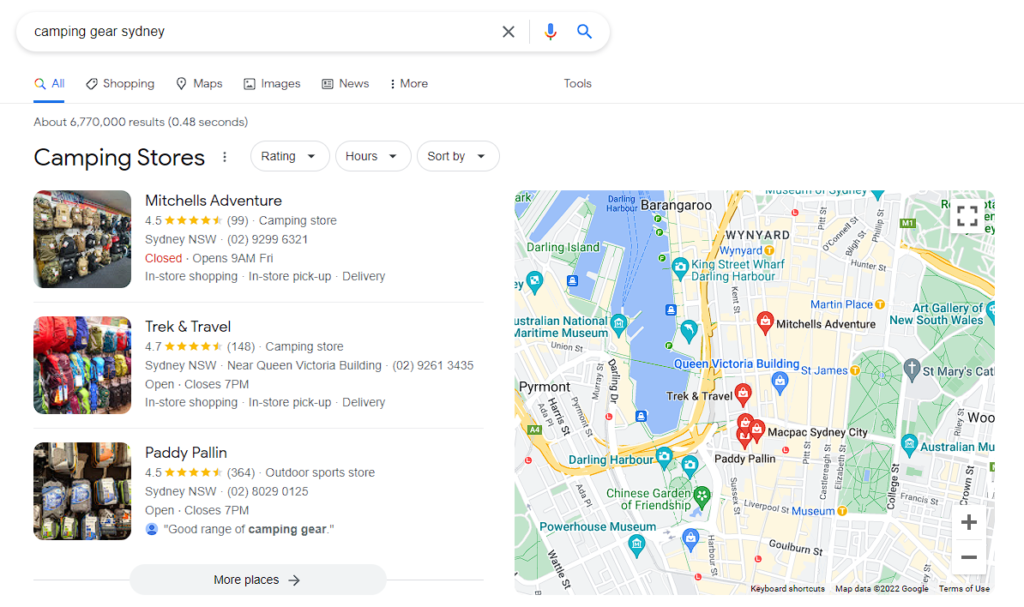The image depicts a Google search results page for "Camping Gear Sydney." Although the Google logo is not visible, the layout is unmistakably similar to a typical Google search interface. At the top, the search bar contains the query "Camping Gear Sydney." The "All" tab is highlighted in blue, indicating the current selection, with other available tabs including Shopping, Maps, Images, News, More, and Tools. The search query yields approximately 6,770,000 results in 0.48 seconds.

The top result is for "Mitchell's Adventure," a camping store that boasts a 4.5-star rating from 99 reviews. The listing includes a phone number, indicates that the store is currently closed, and offers information on in-store shopping, in-store pickup, and delivery options. The accompanying image shows shelves stocked with camping gear.

The second result is "Trek & Travel," another camping store with a higher rating of 4.7 stars from 148 reviews. This listing provides the store's address, phone number, and operating hours, along with options for in-store shopping and delivery. The image associated with this store similarly depicts shelves filled with camping gear.

The third result features "Paddy Palin," an outdoor sports store with a 4.5-star rating based on 364 reviews. This entry also lists the phone number, location, and a review snippet that mentions "a good range of camping gear," highlighted beside a blue circle with a head-and-shoulders icon representing the reviewer. The image shows a close-up of camping gear on shelves.

At the bottom of the search results, a grey rectangle labeled "More places" is visible. On the right side of the page is a map with red pins marking various store locations. The pins correspond to the listed stores such as "Paddy Palin" and "Trek & Travel," with additional locations that are truncated from view in the current image.

Overall, the search results provide a detailed overview of camping gear retailers in Sydney, complete with ratings, reviews, and visual representations of store interiors.